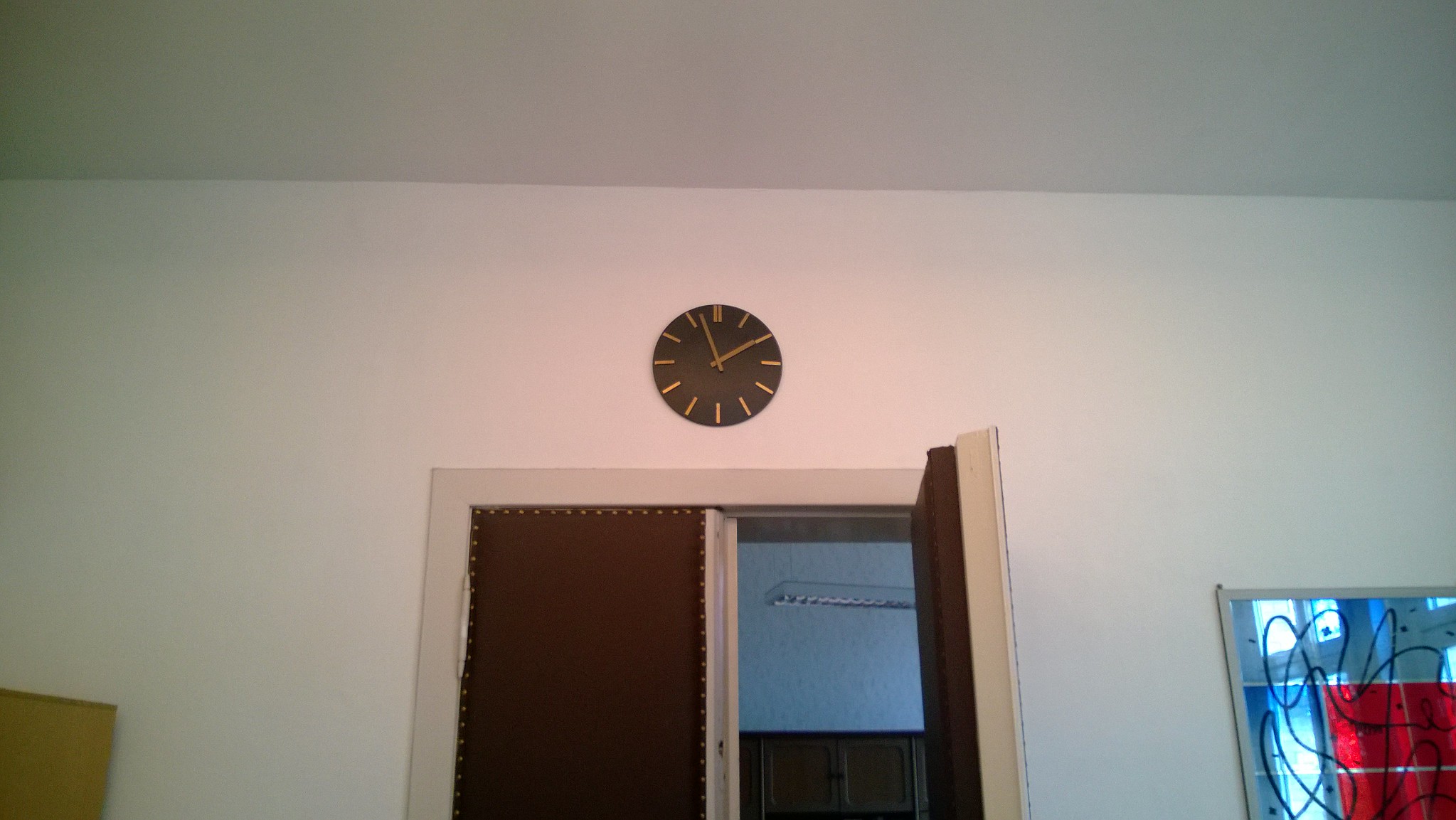The photograph appears to be taken inside a cozy, lived-in home. The ceiling is painted a clean, crisp white, as is the section of wall visible in the frame. A door frame is also prominently featured, constructed with two panels; one side exhibits a rich mahogany wood, while the other is painted white. The door itself is open, revealing an adjoining room. Within this adjacent space, there is a double-sided cabinet in a deep brown hue, positioned beneath a ceiling fan, of which a portion is visible above the cabinet doors.

A clock hangs on the wall, directly facing the viewer. The clock features a dark face, nearly black, with golden hands and numbers that are minimalistic dashes, providing a classic and elegant touch. Off to one side, there is a reflective or decorative piece that resembles lit-up Christmas decor, adorned with vibrant blue and red lights. In the very corner of the photograph, another item is partially visible, distinguishable by its unappealing green color. The scene suggests a warm, eclectic home space, decorated with both practical and festive elements.